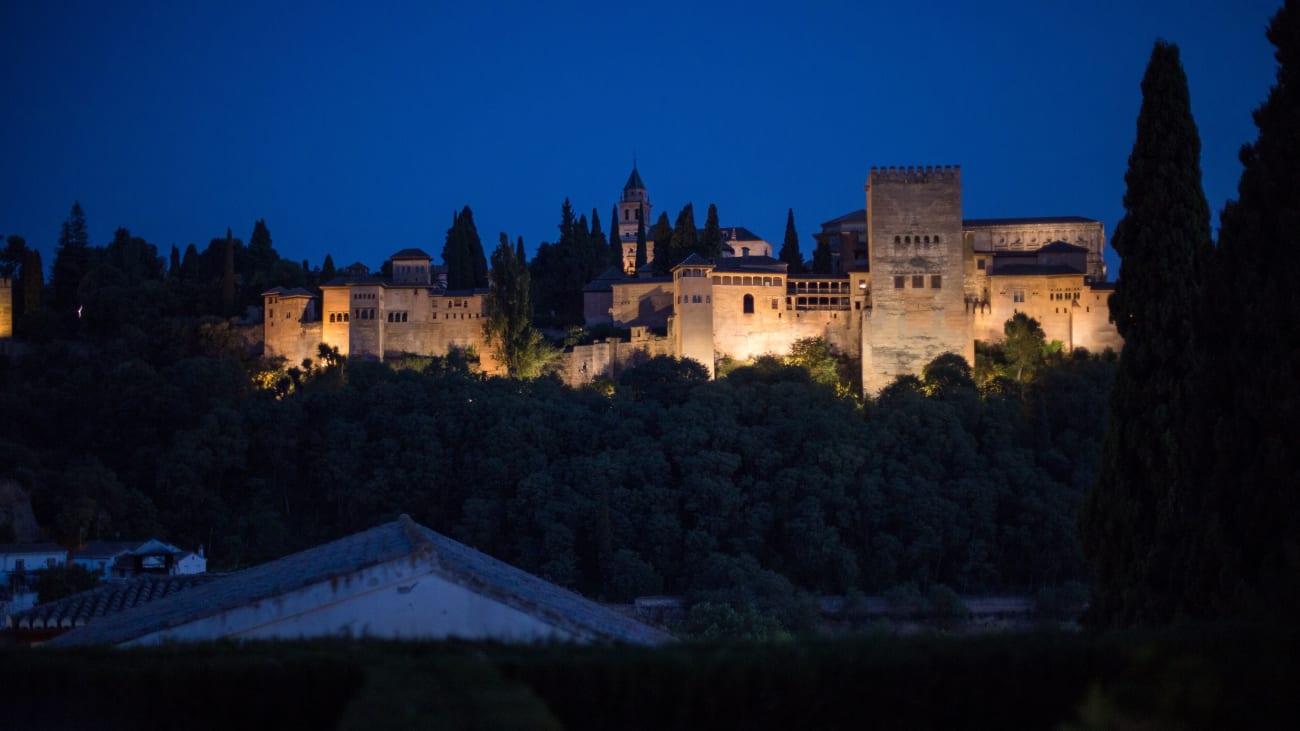The photograph captures a majestic, large castle at night, illuminated by bright white lights from below, casting a warm, golden glow on its beige stone walls. The foreground is adorned with numerous trees of varying sizes, including prominent evergreens on the right side of the frame. At the lower right corner, the edge of a rectangular structure, possibly a swimming pool, is partially visible. The castle's expansive, elongated structure features several towers, including a pointed one at the rear and a flat-topped lookout tower up front. In the dark, starless sky, a deep blue hue sets a tranquil, enchanting backdrop, highlighting the castle's grandeur and its elevated position, possibly on a hill. In the extreme foreground, the arched roofline of another building peeks out at the very bottom of the image.